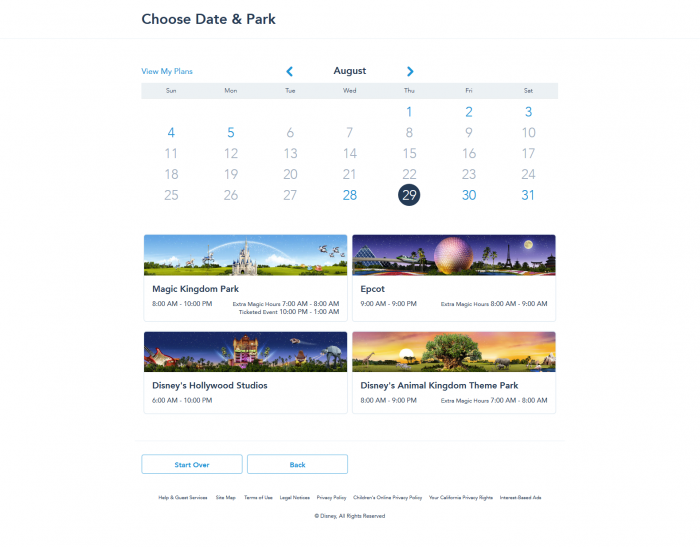This image showcases a detailed view of a Disney-themed calendar interface for planning park visits. In the upper right corner, there is black text reading "Choose Date and Park," and below that, blue text indicating "View My Plans." The header features left and right arrow brackets surrounding the word "August," indicating the current month. The calendar displays dates in August, with some days highlighted in blue and others in gray. The selected date is Thursday, August 29th, highlighted with a dark blue circle and white text.

Below the calendar, there are listed options for different Disney parks along with their operating hours:

- **Magical Kingdom Park**: 8:00 AM - 10:00 PM
- **Epcot**: 9:00 AM - 9:00 PM
- **Disney Hollywood Studios**: 6:00 AM - 10:00 PM
- **Disney Animal Kingdom Theme Park**: 8:00 AM - 9:00 PM

At the bottom of the interface, there are two blue-outlined buttons with blue text offering navigation options. One button reads "Start Over," and the other has the text "SR Back." Finally, the bottom of the page contains typical legal disclaimers, including "Disney's all rights reserved," similar to what is often found on official web pages.